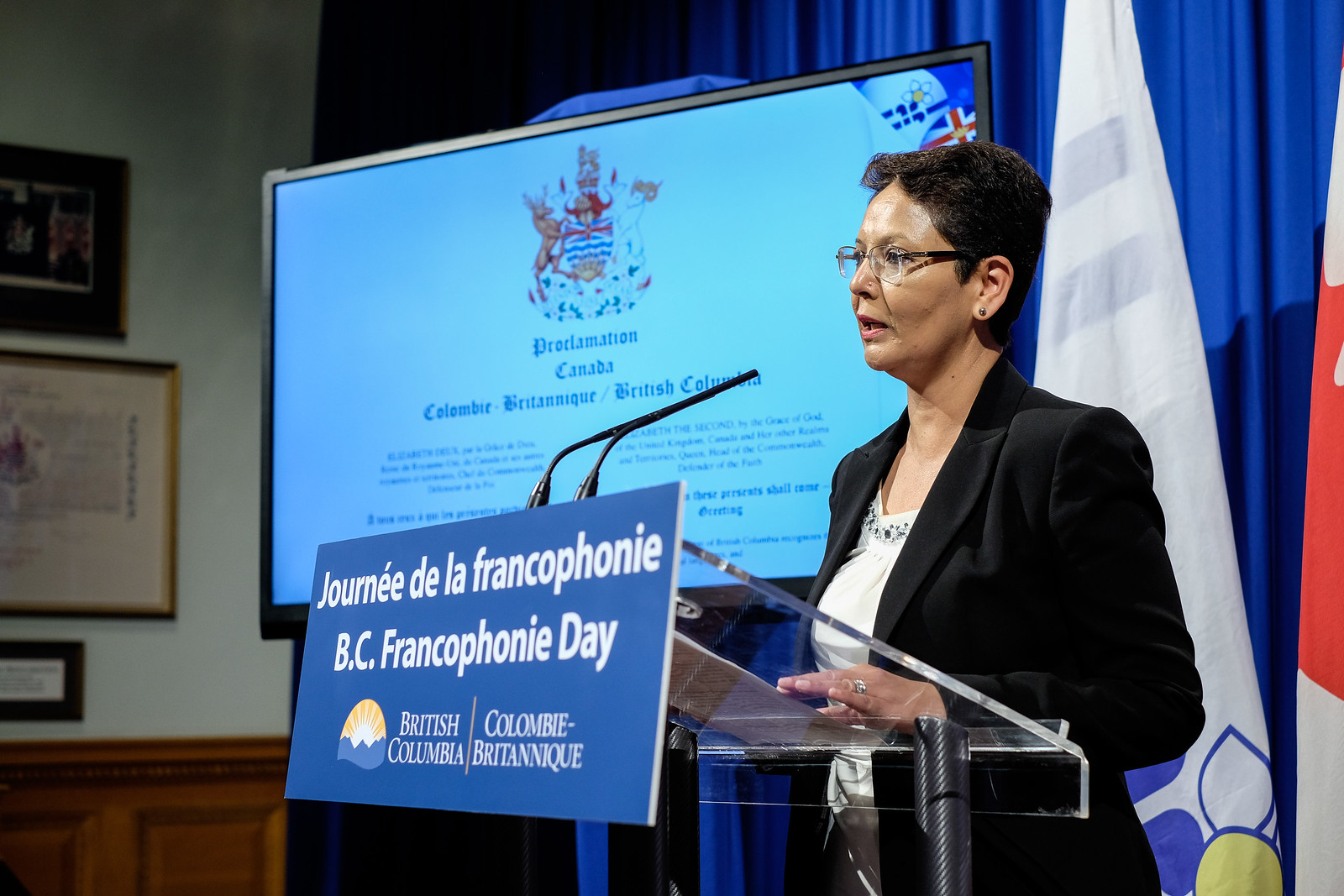A distinguished woman, likely a politician, is delivering a speech at a press conference in British Columbia, Canada. She appears well-prepared and knowledgeable, speaking confidently in French. Her professional demeanor is underscored by her composure and the notes she has in front of her. The background text, also in French, is not fully readable but complements the formal setting. Dressed in a smart jacket, despite a less formal top underneath, she exudes respect and authority. Her hairstyle is neatly done, adding to her strong, independent appearance, which aligns with the persona of a capable and respected political figure.